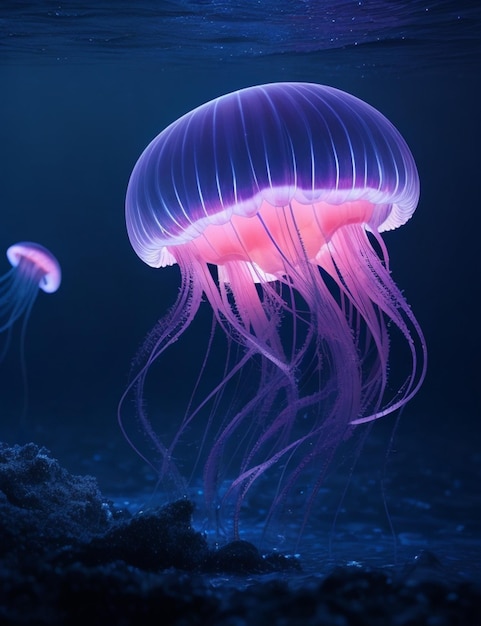The image portrays an underwater scene bathed in deep blue and purple hues, capturing two ethereal jellyfish that appear to be calmly floating near the ocean floor. The larger, prominently placed jellyfish in the center of the image glows brilliantly with a bright pink underbelly and white-striped, purple hood. Its tentacles, which drift gracefully beneath its bulbous body, touch the rocky seabed below. Slightly to the left and in the background, a second, smaller jellyfish, which mirrors the first in appearance, glows softly, adding depth to the scene. Both jellyfish emit a subtle luminescence that gently illuminates the surrounding dark waters and the rocky ocean floor, enhancing the captivating, serene atmosphere of the deep-sea environment.